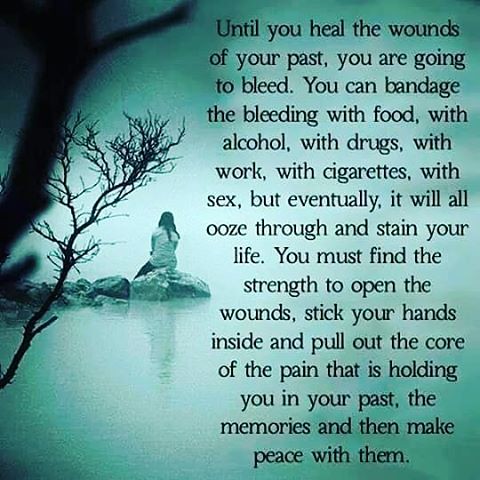The image depicts a woman with her back turned to the camera, sitting on a rock amidst a reflective, green-toned water background. A blurred, black tree branch extends from the top left side of the composition. The woman, appearing contemplative or in despair, kneels on the rock beneath additional boulders. Accompanying the scene, a poignant block of black text reads: "Until you heal the wounds of your past, you are going to bleed. You can bandage the bleeding with food, with alcohol, with drugs, with work, with cigarettes, with sex, but eventually it will all ooze through and stain your life. You must find the strength to open the wounds, stick your hands inside and pull out the core of the pain that is holding you in the past, the memories, and then make peace with them." This evocative and inspirational quote emphasizes the necessity of confronting and healing past traumas to prevent them from continuously affecting one's present life.